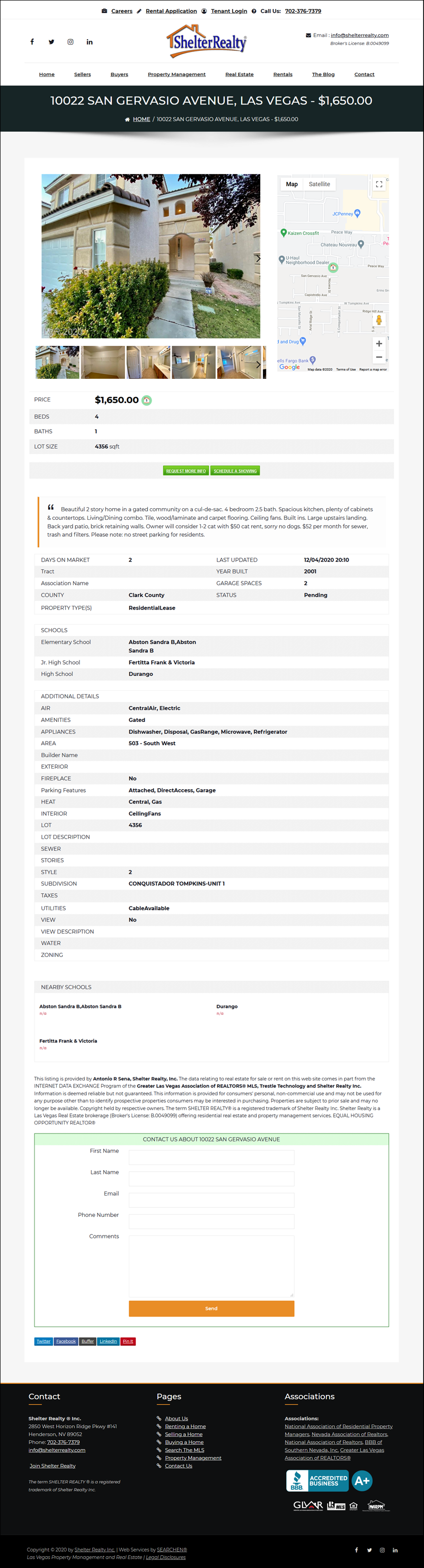This image is a screenshot of a rental application form from the Shelter Realty website, albeit shown in a very small size. At the top, the Shelter Realty logo is displayed with the words "Shelter Realty" over an outline of a house. A navigation menu is present with options such as Home, Sellers, Buyers, Property Management, Real Estate, Rentals, The Blog, and Contact.

Just below the navigation bar, there is a black strip containing the address "10022 San Gervasio Avenue, Las Vegas" and the rental price "$1,650". 

The main content area is divided into two sections. On the left is a large image of the front of the house, and on the right is a map indicating the property’s location. Beneath the large house image, there are several thumbnail pictures available, which likely provide an interior view of the house.

Information about the rental property is detailed there, indicating a price of $1,650, four bedrooms, one bathroom, and a lot size of 4,356 square feet. A descriptive blurb provides additional details about the property, including:

- Days on the Market
- Association Name
- County
- Property Type
- Schools (Elementary, Junior, and High School)
- Additional Features (air conditioning, amenities, appliances)
- Builder Name
- Exterior Details
- Fireplace
- Parking Features
- Heating Type
- Interior Specifications
- Lot Description
- Sewer Type
- Number of Stories
- Architectural Style
- Subdivision
- Taxes
- Utilities
- View and its Description
- Water Source
- Zoning Information

At the bottom of the screenshot, an application form is visible for potential renters to fill out.